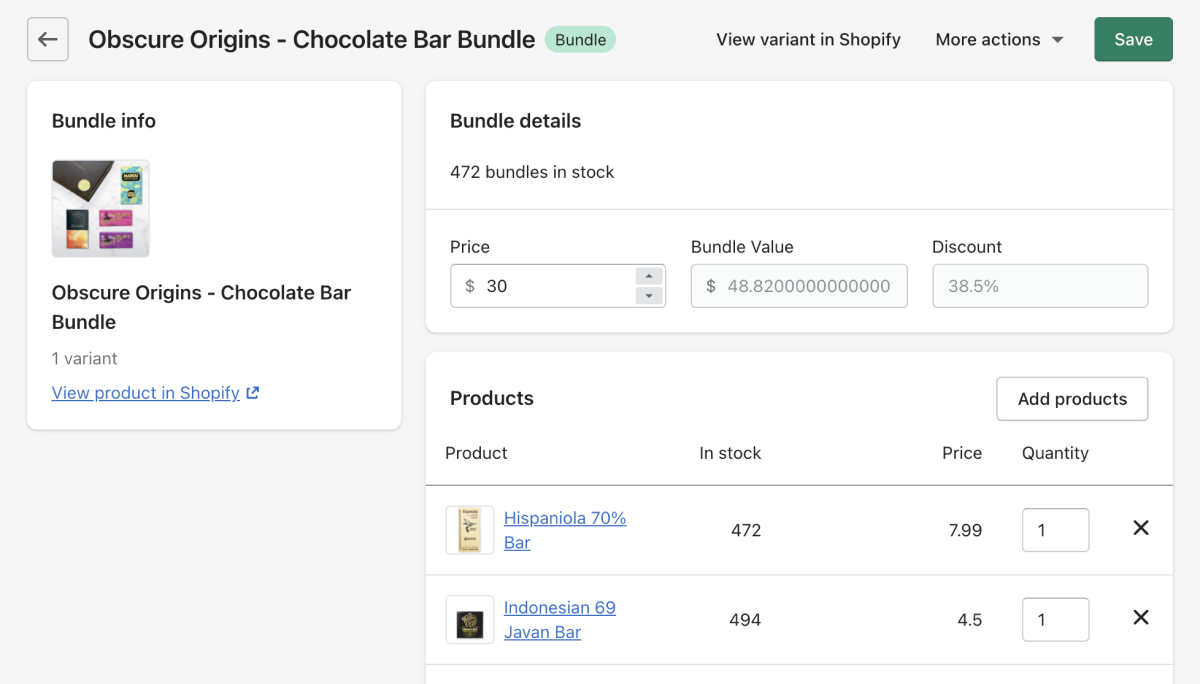The image is a screenshot from a website with a light gray background. At the top of the page, there's a small square on the top left corner featuring a left-pointing arrow. Beside this arrow, black text reads "Obscure Origins - Chocolate Bar Bundle." Below this text, there's a dark green oval with the word "BUNDLE" inside in darker green text. Adjacent to this, the text "View Variant in Shopify" appears, with "Shopify" starting with a capital 'S.' Further along is a "More Actions" button accompanied by a down arrow.

Towards the right side, there is a green button with the word "Save" in white, also starting with a capital 'S.' Moving down the left side of the page, there is a section labeled "Bundle Info," featuring another small square displaying various candies in different wrappings. Below this image, the text reads "Obscure Origins - Chocolate Bar Bundle, One Variant." Underlined in blue, the phrase "View Product in Shopify" appears as a clickable link.

On the right side, there are two white rectangles. The first one is titled "Bundle Details" and lists the following information: 472 bundles in stock, priced at $30 each, with a total bundle value of $48.82, and a discount of 38.5%. 

The second rectangle details the products included in the bundle, along with their stock levels and prices. The first product is "Hyphenolia 70% Bar," with 472 units in stock, priced at $79.99 each, and a quantity of one is specified. An 'X' is located outside this entry. The next product is "Indonesian 69 Javan Bar," with 494 units in stock, priced at $4.50 each, and likewise, a quantity of one is specified, with another 'X' next to the entry.